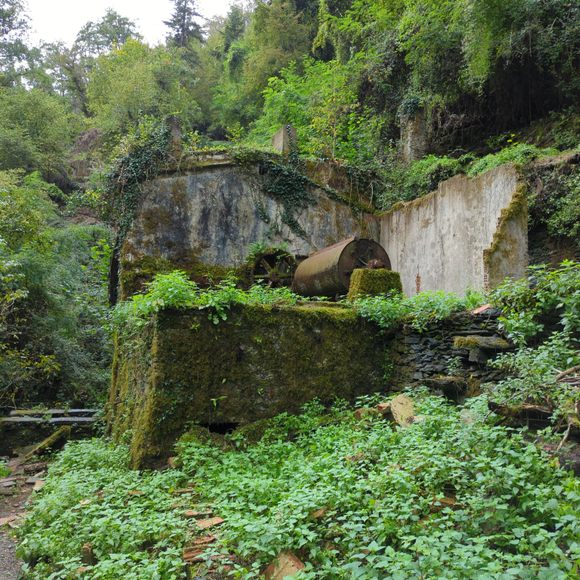The image depicts a verdant outdoor scene with abundant greenery. In the upper left corner, there is a portion of a bright white sky, below which lies a cliff covered in deciduous trees, vines, and scattered branches. Central to the image is an old, partially ruined concrete wall or rock formation, likely the remnants of a building, with its worn stone foundation extending downward. Moss covers parts of this structure, adding to its aged appearance. Dominating the middle of the foundation is a large, rusted, cylindrical barrel or device, positioned at a diagonal angle. Adjacent to this are various bushes, primarily on the bottom right, with a dirt path interspersed with rocks visible on the left side of the image. The overall scene is framed by an overgrown area with numerous plants and trees, creating a vivid depiction of nature reclaiming man-made structures.